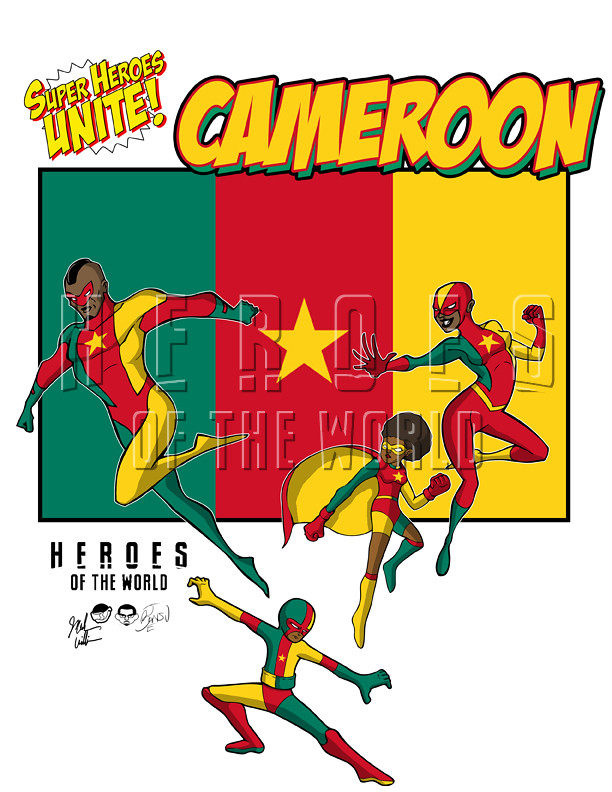The image appears to be an advertisement for a comic book featuring superheroes from Cameroon, titled "Superheroes Unite, Cameroon!" The top of the image prominently displays this title in bright yellow bubble letters designed to grab attention. Below the title is the flag of Cameroon, which has three vertical stripes—green on the left, red in the middle with a yellow star, and yellow on the right. The flag also features a watermark saying "Heroes of the World."

In the foreground, there are four superheroes—a man positioned in front of the green stripe, a woman in front of the yellow stripe, a young girl spanning the red and yellow sections, and a young boy striking a fighting pose below. They all have darker skin tones, suggesting they are of African descent, likely African-American. Each character is dressed in costumes that mirror the colors of the flag, featuring green, red, and yellow, with a prominent yellow star on their chests. The bottom left of the image includes black lettering that says "Heroes of the World," along with the artist's signature.